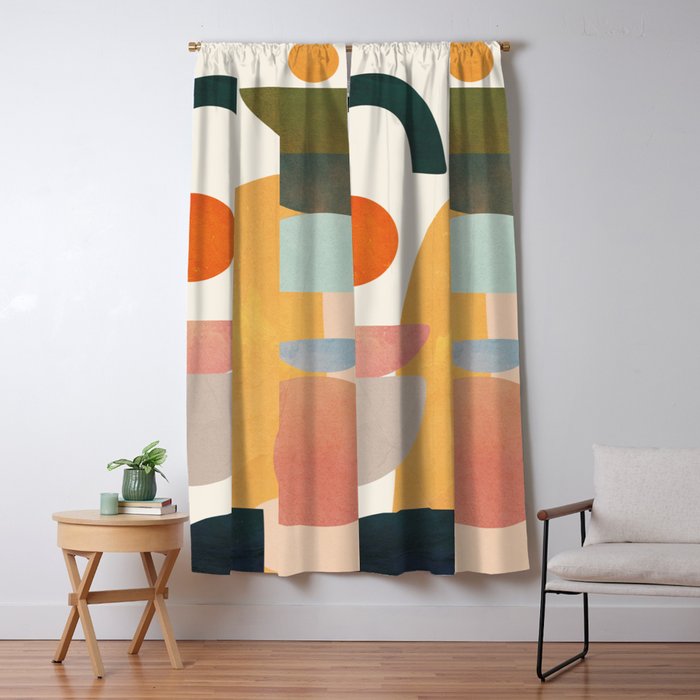This image features a set of window curtains with a multicolored abstract pattern consisting of various shapes, including tall skinny arches, blobbish circular shapes, half circles, and ovals. Each shape in the pattern sports a different color, such as orange, pink, taupe, gold, sky blue, army green, evergreen, gray, mauve, and black, all beautifully juxtaposed against a light creamy white background. The curtains, which are identical in design, are depicted hanging from a brown curtain rod mounted on an off-white or gray wall. A notable feature is the white stitching along the hem at the top of the curtains, which is prominently visible. These curtains are relatively long rather than wide, and the image captures them centered in the frame with light filtering through, highlighting the intricate design. The floor beneath the curtains has a subtle gray tone, adding to the overall harmonious color palette of the scene.